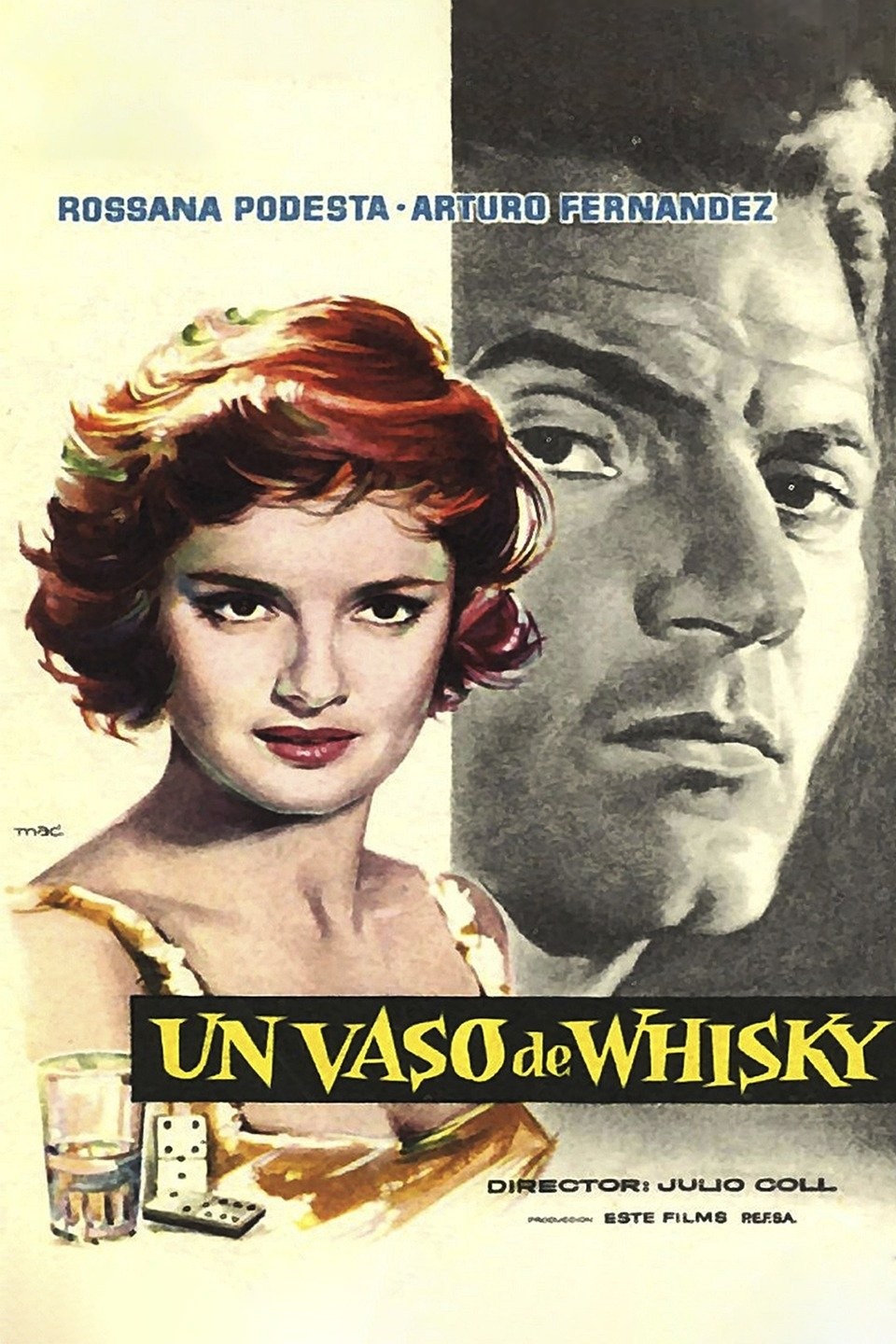The vintage movie poster prominently features two actors: Rosana Podesta and Arturo Fernandez. On the left side, there is a color illustration of Rosana Podesta with bright red, short hair that sweeps to the right, wearing lipstick and a low-cut, golden-yellow top. In front of her, there is a small glass of what appears to be whiskey and two white dominoes with black circles. The right side of the poster displays a close-up black-and-white photograph of Arturo Fernandez, characterized by his dark hair swooped back, thick dark eyebrows, and a cleft chin, with a mysterious, serious expression. The background behind Rosana is off-white. The actors' names are written across the top in blue lettering, reading "Rosana Podesta · Arturo Fernandez." Below their images, in a black bar with yellow lettering, is the title "Un Vaso de Whiskey" and beneath that, it states "director Julio Cole."